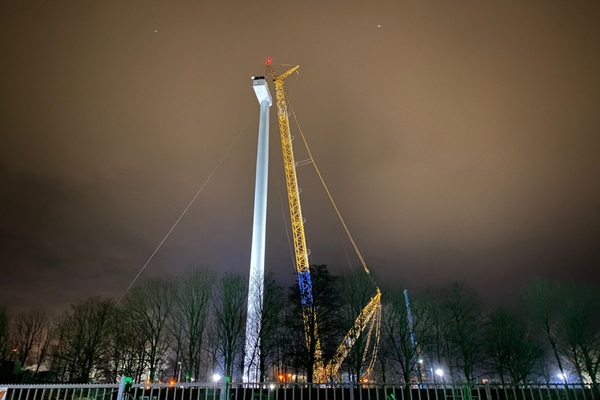The image captures a nighttime scene in what appears to be an urban or industrial area, potentially in the US or South Korea. Dominating the scene is a tall crane illuminated with hundreds of vibrant LED lights in yellow, blue, and green. Adjacent to the crane is a tower-like structure with a platform at the top, possibly under construction with the aid of the crane. This tower is supported by scaffolding, steel cables, and struts for stability. At the very top of the tower, a red light possibly blinks against a murky brown evening sky. Below, a segmented gray metal fence borders the area, with light vegetation suggestive of a park or an industrial green space through which construction equipment and more lights are visible. The scene is intricately lit, juxtaposing the towering structures against the dark night sky, creating a visually compelling industrial tableau.